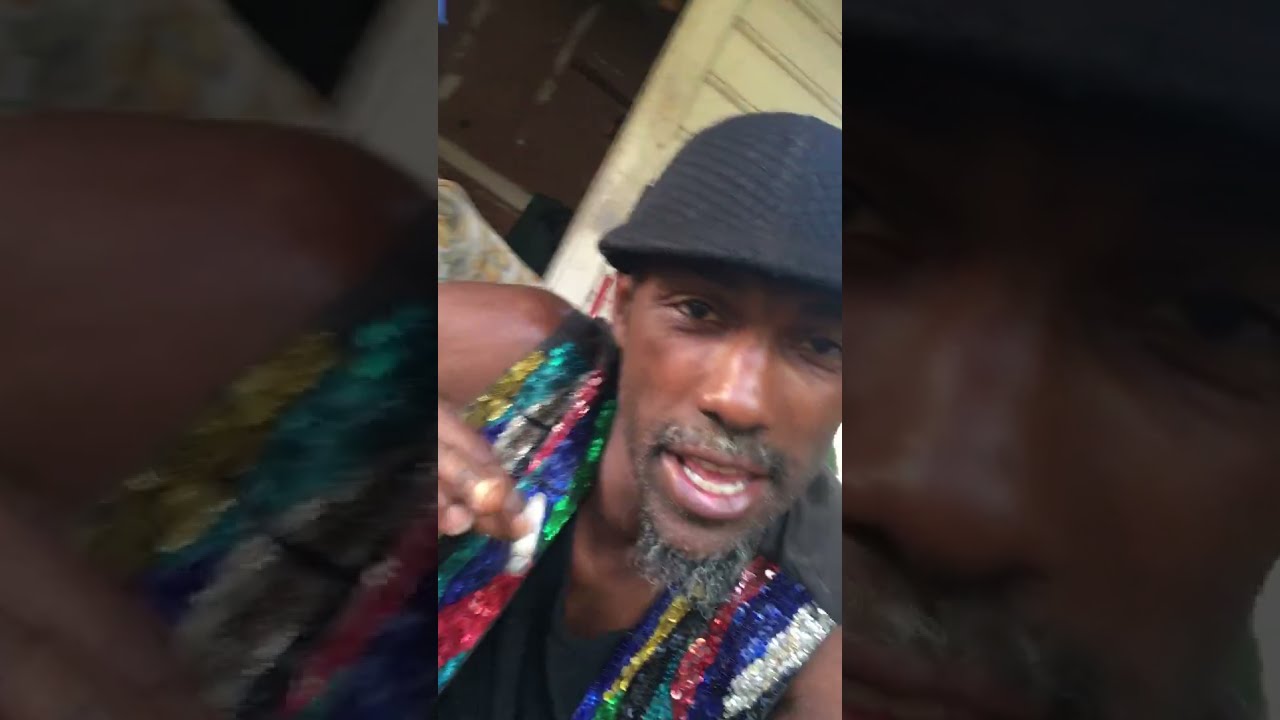The image captures a middle-aged African-American man taking a selfie while seated in a tan-colored chair with floral patterns, on a house's patio. He is positioned in the center of the frame, flanked by thick black borders on both sides of the image. The man is wearing a distinctive black hat, akin to a horse riding cap but with a more pronounced brim. His facial features include a mustache and a goatee flecked with gray hairs, and he's looking directly at the camera with a slight smirk and slightly open mouth, revealing both his top and bottom teeth. He is dressed in a striking black vest adorned with sequins in blue, yellow, green, black, light blue, and red, over a black sleeveless tank top. The background includes a red broom handle with a black end cap and a window set into the dirty white paneling of the house. An open door is visible to the left, emphasizing the outdoor setting.